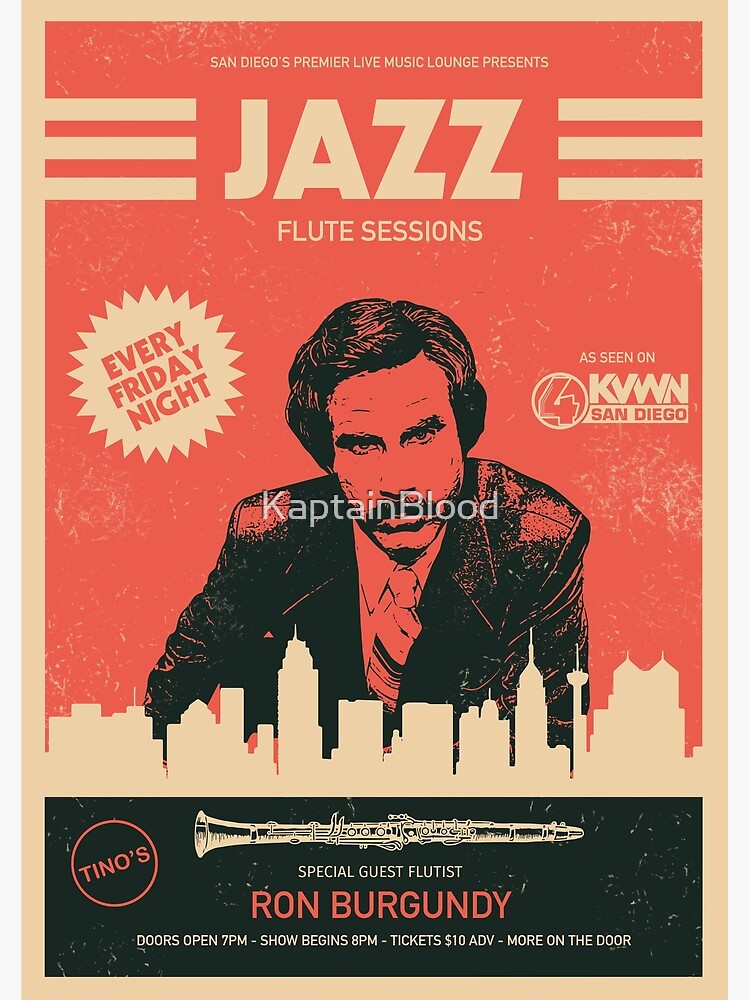This is a vibrant advertisement poster predominantly in shades of red, yellow, and black, promoting San Diego's Premier Live Music Lounge's Jazz Flute Sessions. The top of the poster announces, "San Diego's Premier Live Music Lounge Presents Jazz Flute Sessions Every Friday Night." Below this text, a black drawing of a man with a side part and a mustache, dressed in a suit jacket and tie, captures attention. This character, Ron Burgundy, the special guest flautist, hovers over a pale yellow cityscape of San Diego. Beneath the cityscape is a yellow and black illustration of a flute. Details include "Doors open 7 PM, show begins 8 PM, tickets $10 ADV, more on the door." The middle of the image also features a watermark that reads "Captain Blood," noting the unique spelling with a "K." As seen on KVWN San Diego, this fictional jazz flute session promises an entertaining evening.